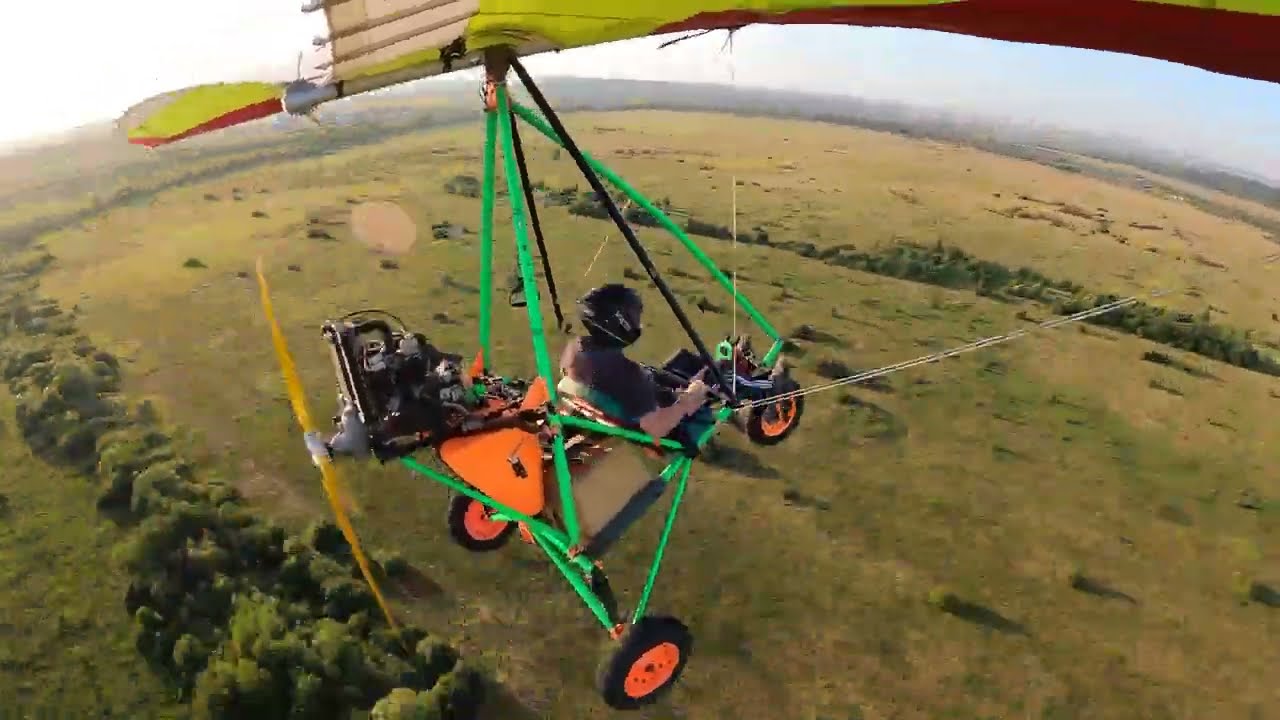In this vivid photograph, a man is seen soaring about 50 feet above an expansive, green and yellow field, utilizing a self-made airborne contraption. The device, which resembles a hybrid between a tricycle and a glider, features a vibrant yellow and brown wing structure supported by three triangular beams. The contraption is predominantly green, with the seated man positioned at the front, donning a gray t-shirt and a black helmet. The rear houses a small motor equipped with a yellow propeller, helping to sustain flight. The three-wheeled base, reminiscent of a tricycle with rubber tires and orange accents, also shares visual similarity to parts from a dirt bike or lawnmower. Below, patterns of rows of trees interspersed with open grasslands extend toward the horizon, where the sky transitions from a serene white to blue. The photograph captures the striking image of the glider navigating the sky, evoking a sense of innovation and adventure.